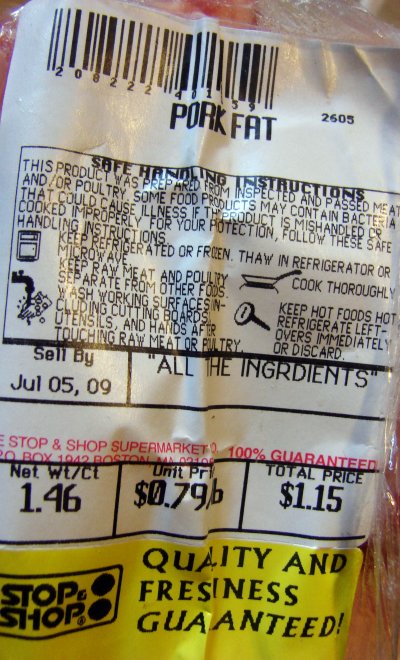The image features a detailed label for pork fat from the grocery store Stop & Shop. At the top left, there is a barcode with the numbers "208222 401159" and "2605". Beneath the barcode, the label prominently states "Pork Fat" in black type on a white background. Below this, there is a rectangular section containing "Safe Handling Instructions," advising that the product was prepared from inspected and passed meat or poultry, and warning of potential bacteria if mishandled or improperly cooked. Visual icons such as a thermometer and a frying pan illustrate proper handling techniques. Further down, the label displays a sell-by date of July 5th, 2009, alongside a misprinted "INGRDINTS" heading. Following this, the net weight of the product is listed as 1.46 pounds, with a unit price of $0.79 per pound leading to a total price of $1.15. At the very bottom, a yellow band declares the grocery store name "Stop & Shop" with the assurance "Quality and Freshness Guaranteed."